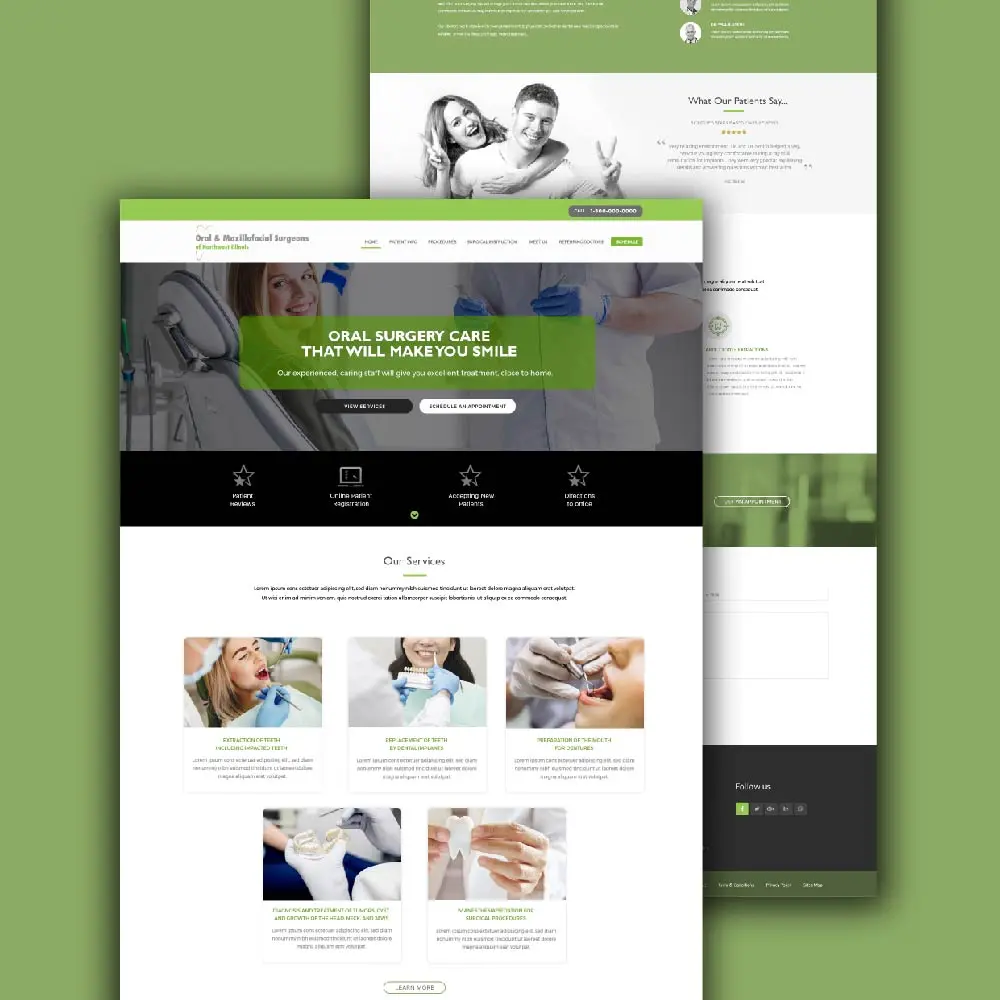The screenshot displays a website dedicated to oral and maxillofacial surgery services. The background is a light green color with two overlapping fields. The partially covered field features an image of a man and a woman making peace signs with a caption relating to partner testimonials and reviews.

In the foreground, a more prominent section includes a header above a color photo of a woman smiling while seated in a dentist's chair. Beside her stands a man wearing a white coat and blue surgical gloves. The text "Oral surgery care that will make you smile" is displayed against a green overlay, though some text remains partially obscured. Below this, a black-and-white button is present but unreadable due to partial greying out.

Further down, a black bar with three stars and another indistinct rectangular element are positioned above a section titled "Our Services." This section comprises five images: three at the top and two below. The top images depict women undergoing oral inspections by a professional. The bottom images feature someone holding dentures and another holding a model of a large tooth.

Despite some text being unreadable, the overall design conveys a welcoming and professional atmosphere tailored to oral and maxillofacial care.